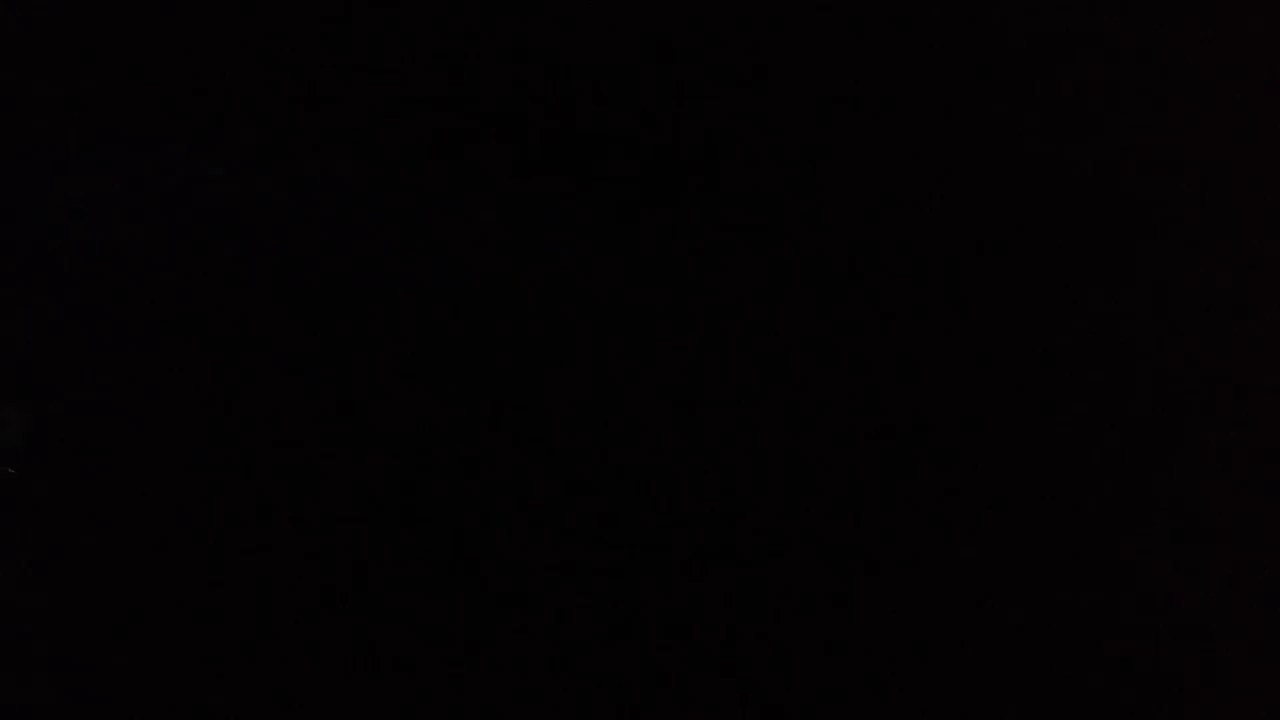The image is a solid black rectangle, entirely devoid of light, detail, or objects. It is uniformly pitch black throughout, with no variations in shade or texture. There are no discernible elements, positions, or text, making the image appear like a black hole or a blank screen. The darkness is consistent and unbroken, suggesting either an incomplete loading or an intentional choice for the image to be entirely black.